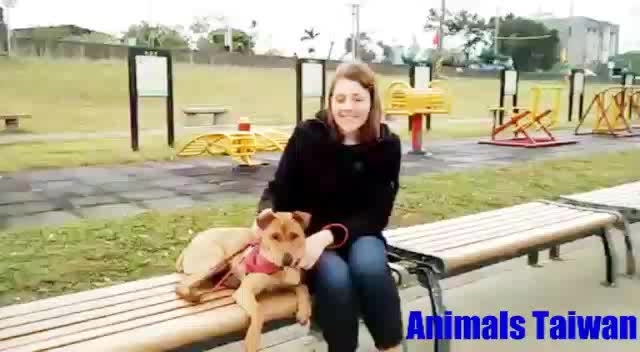This outdoor photograph captures a woman and her dog seated on a wooden bench with metal legs in an urban park setting. The woman, dressed in a black long-sleeved shirt and blue jeans, has brown hair and a subtly smiling face, with one eye appearing closed. Her dog, a small to medium-sized brown dog, sports a bright red bandana around its neck. In the backdrop, there is a series of concrete benches without backrests, a grassy area, and an obstacle course—likely designated for dog activities—with some indiscernible signs. The park extends to show a large green field, residential houses, and a commercial building. A stop sign and various walkway features, including some play structures possibly for children, are also visible. The scene is unified by the "Animals Taiwan" caption in blue text situated in the bottom right corner of the image.